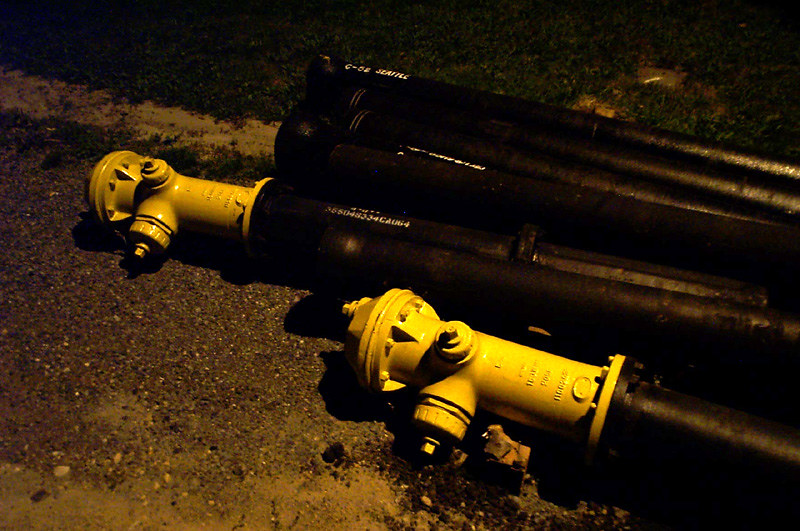In this nighttime photograph, two yellow fire hydrants are laying horizontally on a dirty gray street surface, accompanied by several pipes that are not yet installed. The hydrants, which have various attachments for connecting hoses, are placed on a road that features a mix of sand, stone debris, and gravel. Alongside the street, there's a white painted line marking the boundary between the road shoulder and a small patch of grass. The background includes some curbing that lines the grassy area, indicating this scene is likely near a roadside. The image captures the preparation stage for the installation of these hydrants and their associated pipes.